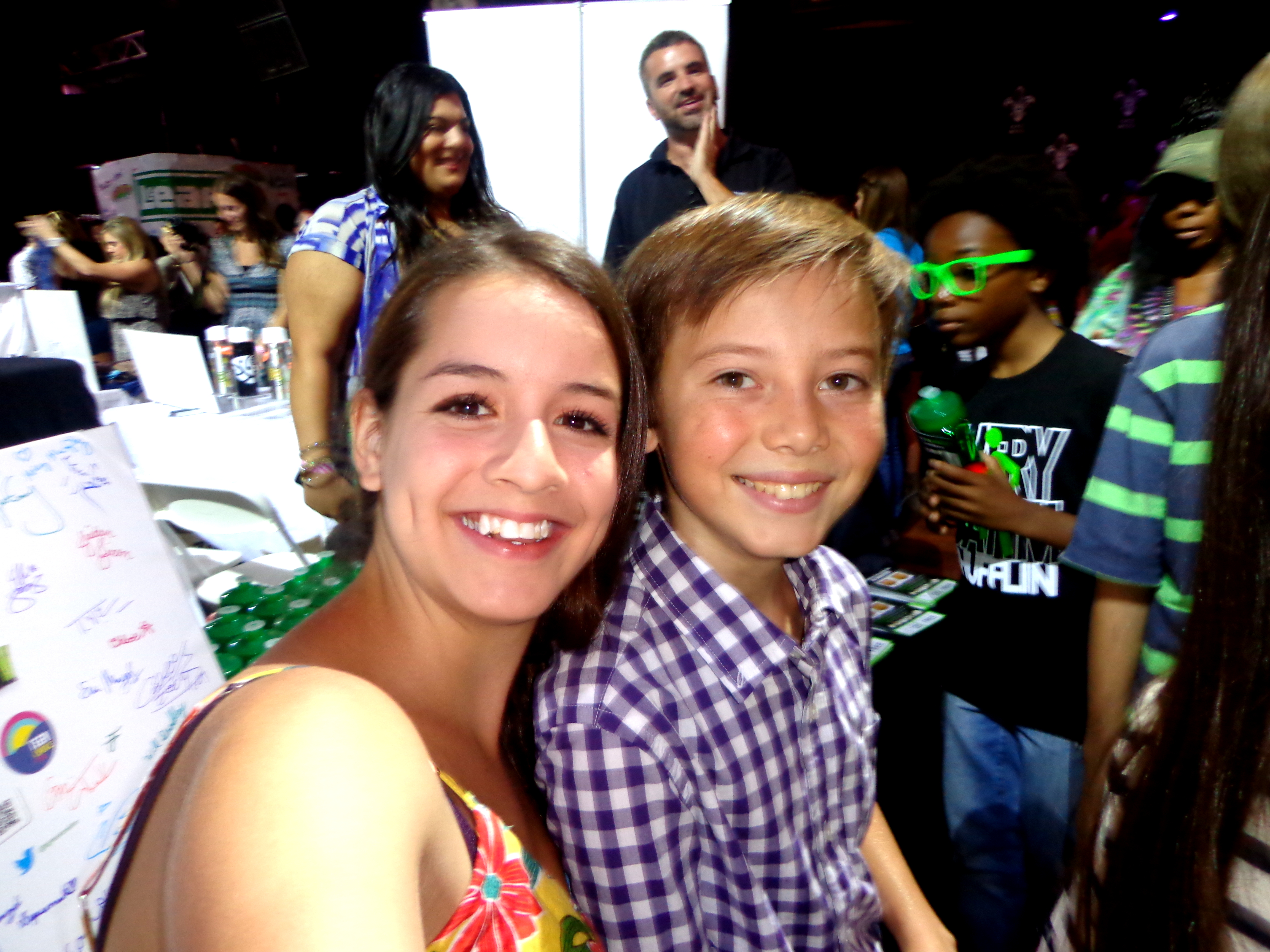In the foreground of this vibrant photograph from an indoor event, a young woman, possibly a teenager or young adult, stands out with her cheerful smile. She is dressed in a thin-strapped, sleeveless white top adorned with red and yellow flowers. Beside her, on the right, a young boy, around 8 years old, shares her joyful expression. He sports a blue button-up polo shirt. Behind them, over the woman’s shoulder, a whiteboard teeming with multicolored handwritten autographs adds to the lively atmosphere. The background reveals a bustling scene with numerous people milling around, suggestive of a convention or trade show. Among them, a distinct figure is a black boy wearing striking bright green glasses, adding a splash of color to the crowd. A table is also visible amid the sea of attendees, further indicating the busy nature of the event.